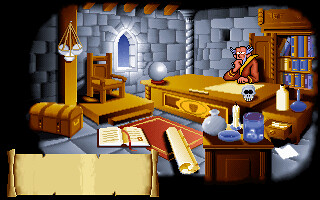This detailed image appears to be a screenshot from a retro point-and-click adventure game with a cartoonish, 2D aesthetic typical of early 90s DOS games. The scene is set inside a castle room with a stone wall backdrop featuring both light and dark gray stones. The foreground prominently displays a well-organized, elaborate setting suggesting a puzzle-mystery game environment where players receive instructions and solve tasks.

In the lower left corner of the image, there's an open, landscape-oriented scroll that appears to be blank, hinting that text is about to appear to provide guidance. Another scroll, also tan with slightly darker edges, lies on the floor near an open book. This book has a red ribbon bookmark, small brown text, and a red symbol on the right-hand page.

At the center of the scene is an aged individual with thinning gray hair, accentuated by blue-gray strands around his head and beard. He is seated in a large brown chair, wearing a brown robe with gold neck accents. The man sits at a large light gray desk adorned with a gray orb resting on a maroon saucer, a tan paper, and a tan rectangular piece. The desk is surrounded by various objects, including a bookshelf behind him filled with blue, green, and brown books, and a skull with black eyes and partially black teeth on the right side edge of the desk. To the right of the large desk, an open drawer reveals more items, and beside it stands a cylindrical blue piece with lighter blue accents, next to a fat vase tapering into a fluke, colored in mid and light gray.

A red rug with gold embroidery lies in front of the desk, enhancing the room's regal atmosphere. In the background, against the stone wall, is a light gray pillar with a three-walled light fixture and a treasure chest that is ornately decorated with orangish-brown hues and darker brown locks. There is also a small window tapering into a triangle at the top, allowing white light to emanate into the room.

Together, these elements create a detailed, immersive scene that invites players to engage in solving mysteries and following the instructions provided within the game.